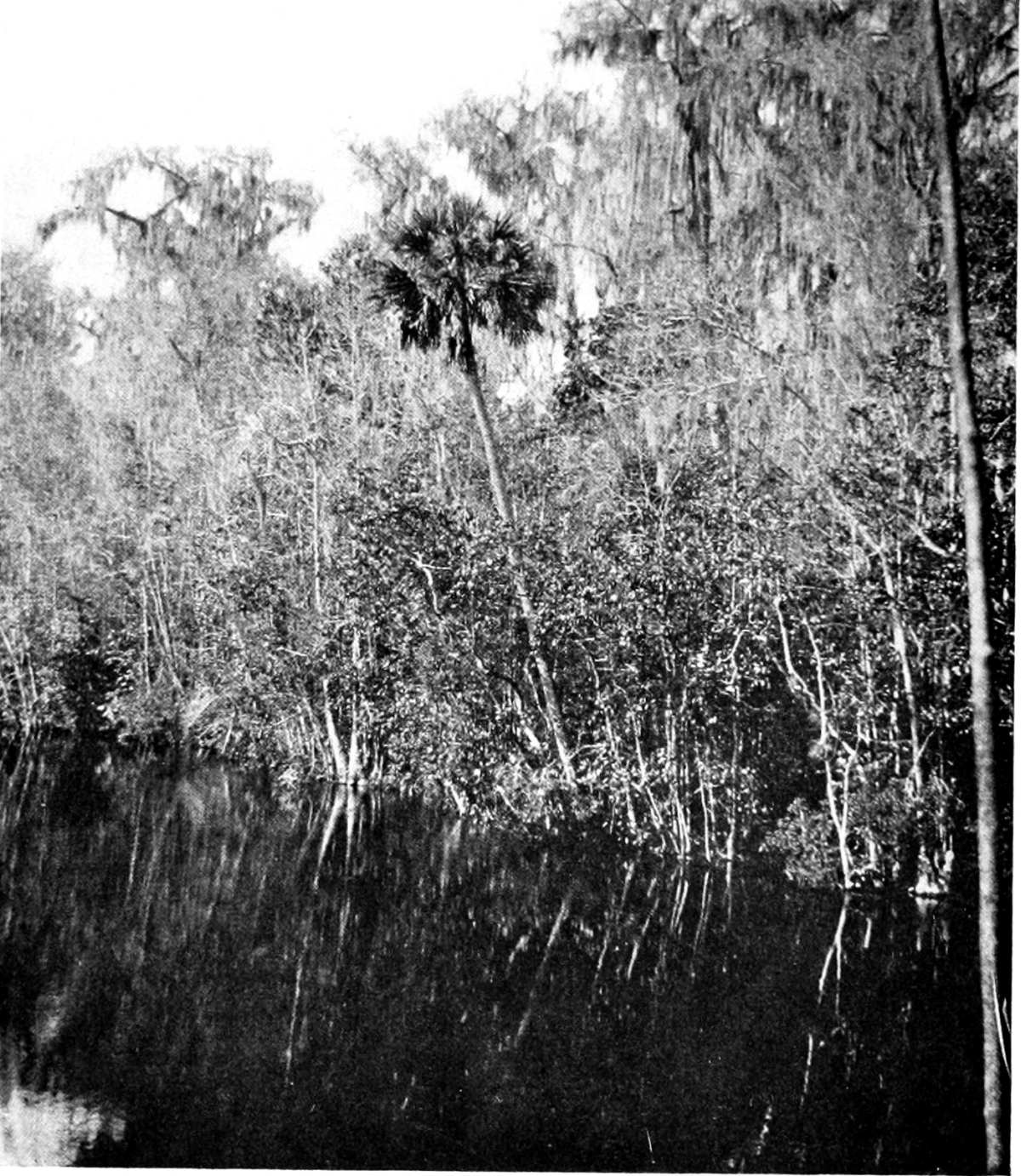This black and white photo captures a serene and uninhabited stretch of natural wilderness that evokes feelings of the dense, untouched swamps found in parts of the southeastern United States. The scene is centered around a gently flowing body of water, possibly a lake or river, with numerous trees surrounding it. A particularly prominent palm tree leans precariously over the water, appearing as if it might soon topple in. The water is calm, reflecting the untouched beauty around it. Surrounding the water are trees draped in moss and undergrowth composed of dense bushes and branches, creating a habitat resembling a mangrove or rainforest. With the sun casting its light subtly across the scene, the image emphasizes the raw and untamed glory of nature, filled with an array of grayscale hues that accentuate the tranquil yet wild environment. No human presence disturbs this natural setting, and the photograph captures the sheer abundance of vegetation, highlighting trees that vary in their shades of gray, interspersed with darker palm leaves. This detailed snapshot of nature in its full, unspoiled glory is strikingly peaceful and immersive.